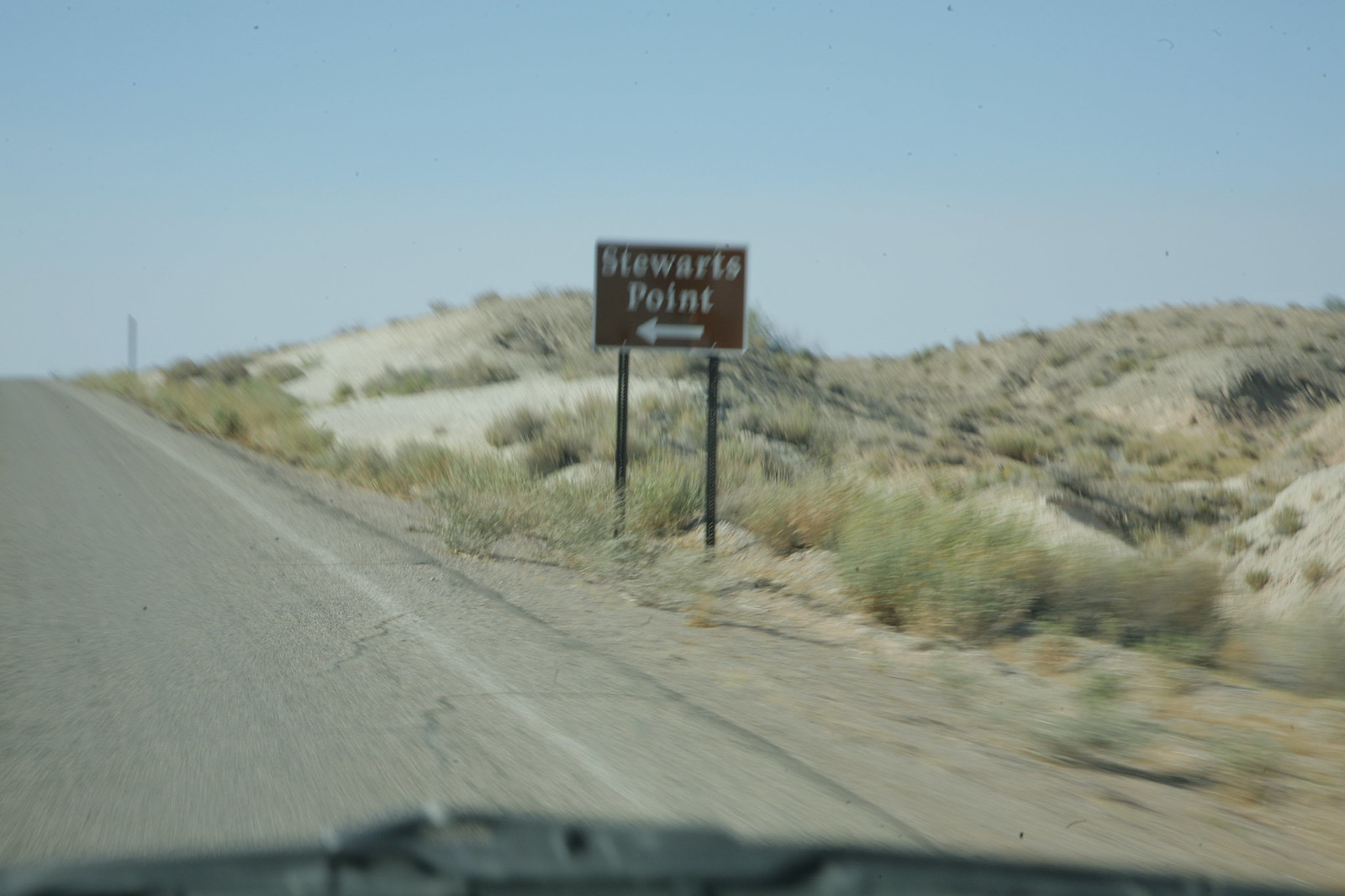The photograph, taken from inside a car, captures a view of a road scene through a slightly out-of-focus car hood or window edge at the bottom. The left half of the image is dominated by a gray asphalt road, while the right half showcases a dry, sandy area featuring sparse tufts of grass. The sand is light beige, and the grass—muted green with tinges of yellow—adds a touch of color to the arid landscape. Centrally positioned in the photograph is a prominent brown sign that reads "Stewart's Point," with an arrow directing to the left, indicating a nearby destination.